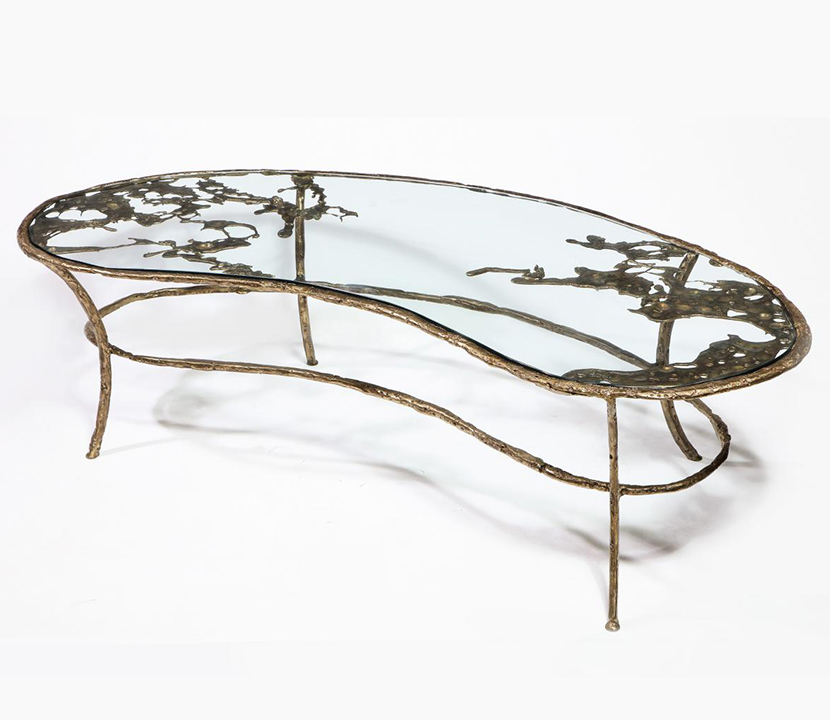This image features an ornate, kidney bean-shaped coffee table that appears to be handcrafted. The table has a glass top with potential metal filigree work embedded within or underneath the surface, giving it an intricate and organic appearance. The metal structure, possibly wrought iron or a bronze-like material, features a brownish bronze hue with a golden, coppery rim. The four arced legs connect to an under ring that mirrors the table's shape but provides no additional shelving. The table's elaborate design includes decorative elements spreading out from the legs and seems to be captured from above, set against a stark white background.